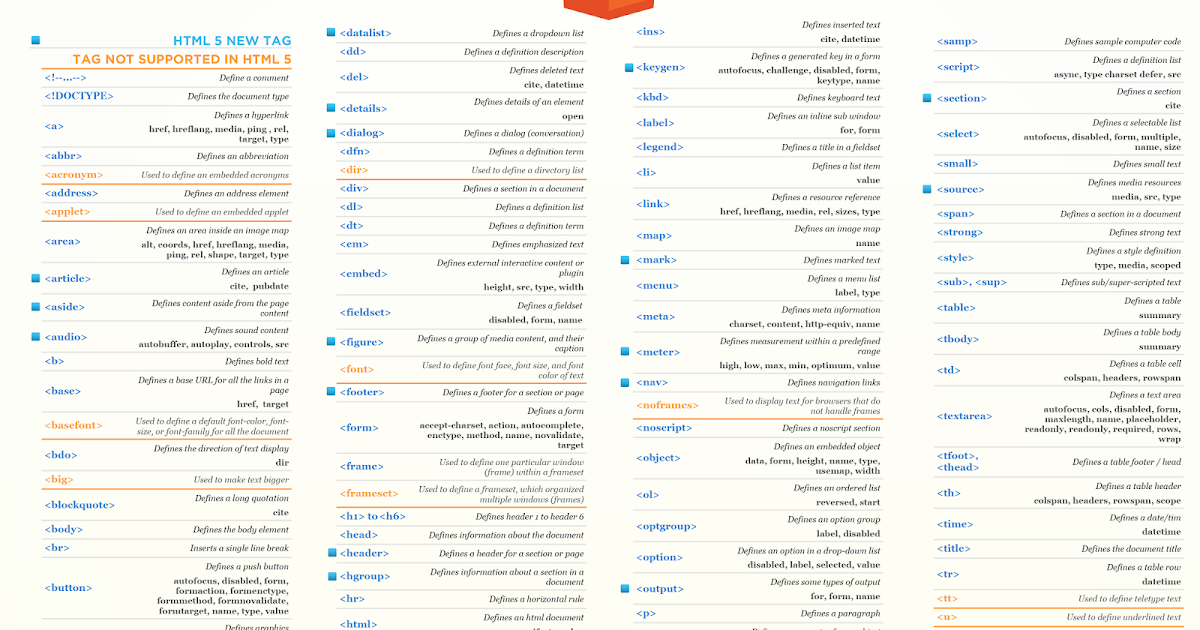A comprehensive reference table is presented, filled with columns of essential HTML5 tags and their descriptions. At the top of the first column, a small blue box sits to the left, juxtaposed with "HTML5 NEW TAG" written in all caps and blue on the right. Below this heading, an orange text denotes "new line tag not supporting HTML."

This table lists various HTML5 tags, each associated with specific keyboard commands for different functions:

- The first entry includes a combination of symbols like left arrows, exclamations, hyphens, and periods, meant for defining a comment.
- The subsequent entry features a different set of symbols, indicating it defines a document type.
- Further down, a tag "<a>" is shown, which defines a hyperlink, accompanied by attributes such as "href," "media," "ping," "rel," "target," and "type" in bold.
- Another tag, "<abbr>", is used for abbreviations and acronyms, specifying how to embed these elements.

This pattern continues throughout the table, delineating various HTML5 tags and respective functions in an organized manner. The background of the table is a beige or off-white color, providing a neutral canvas for the information.

In the middle of the second or third column, a conspicuous red pentagon shape points downward, likely marking a particular section of interest. Tags that are supported are highlighted in orange. Blue text is predominantly used for tag descriptions, with occasional orange text, and each command's meaning is italicized and typically bolded. Orange lines sporadically run through the table to delineate sections further, enhancing readability.